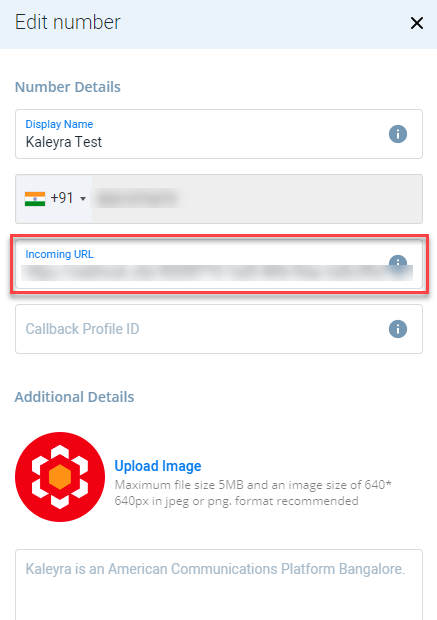This screenshot captures a phone book or contact entry form on a mobile device, designed for inputting and editing someone's contact details. At the top, there is a light blue banner displaying the title "Edit Number" accompanied by a black 'X' icon on the right, suggesting an option to close the form.

Beneath the banner, the section labeled "Number Details" includes several fields. The first field is "Display Name," filled in with "Kaliera Test," and next to this field is an eye-in-a-circle icon, likely providing additional information or options.

Following the display name, the "Phone Number" field is visible, marked by a national flag and the country code "+91," with the actual phone number grayed out and not visible.

The next field, enclosed in a red outline, is labeled "Incoming URL" and also grayed out, indicating that the content is either hidden or not editable. Below, the "Callback Profile ID" field remains blank, displaying only the field name without any input.

Toward the bottom of the form, there is a section labeled "Additional Details," alongside a round icon with a flower in it. This section includes an "Upload Image" option, presumably allowing the user to attach a picture to the contact entry.